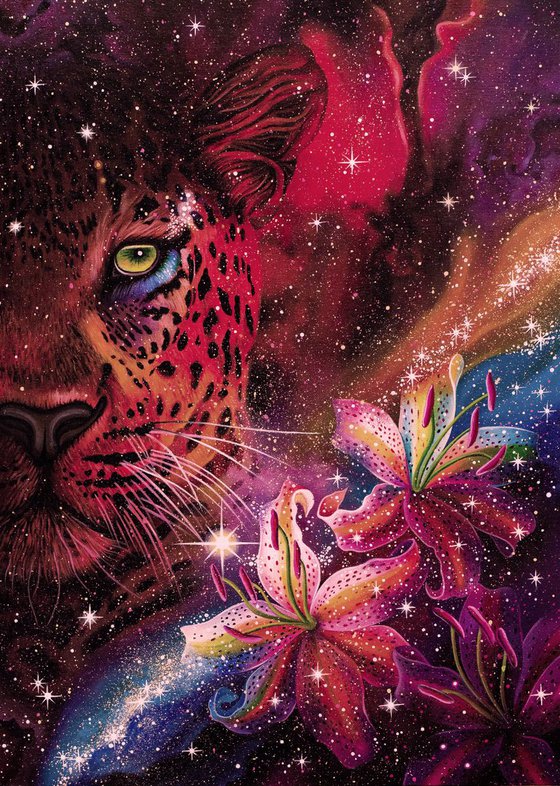This vibrant, psychedelic painting features a mesmerizing scene blending the natural world with cosmic elements. Dominating the upper left portion of the artwork is the striking face of a leopard or jaguar, rendered in an array of colors—primarily orange with black spots, its eye a piercing green with a black iris, and a bluish-purple area beneath it. Gazing directly at the viewer, this creature captivates with its intense presence. The background of the painting is a swirling galaxy, including the Milky Way, adorned with stars of various sizes and clusters, adding depth and a sense of the infinite to the scene.

In the bottom right corner, an assortment of flowers bursts into view, featuring vivid hues of orange, purple, yellow, blue, and green, their colors echoing the nebula's rich palette of red, magenta, pink, and orange. Their pink stems and colorful petals stand in contrast to the starry expanse. Central to the composition and bridging these two elements, the largest star shines brightly, drawing the eye and unifying the celestial and botanical aspects of the artwork. The overall effect is a stunning, otherworldly display that combines the wild beauty of nature with the mysterious allure of the cosmos.